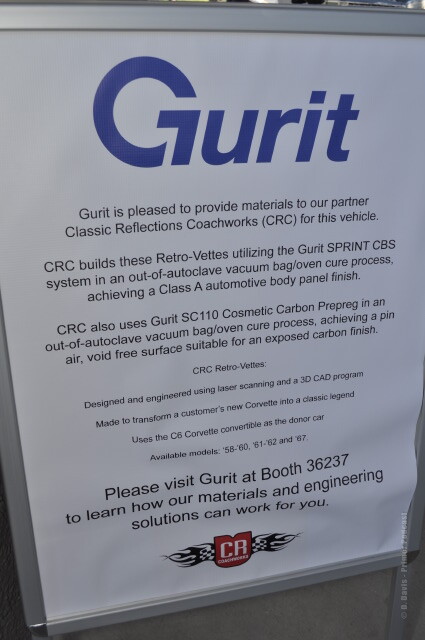The image shows a sign mounted on a grayish wall, framed by a gray border. At the top of the sign, in distinctive blue lettering, it reads "Gurit" (spelled G-U-R-I-T) in a unique font. The sign indicates that Gurit is delighted to provide materials to its partner, Classic Reflections Coachworks (CRC), for their vehicles. This partnership involves CRC utilizing the Gurit Sprint CBS system in an out-of-autoclave vacuum bag/oven cure process to achieve a Class A automotive body panel finish. Additionally, CRC employs Gurit's SC110 cosmetic carbon prepreg in a similar out-of-autoclave process to achieve a pin-air, void-free surface suitable for an exposed carbon finish. The sign details that CRC builds retro vets, designed and engineered using laser scanning and 3D CAD programs, converting new Corvettes into classic legends with models available from '58 to '60, '61 to '62, and '67. It invites attendees to visit Gurit at booth 36237 for further insights into their materials and engineering solutions. At the bottom, the sign features a logo depicting a red shield with black and white wings extending from each side, and the letters "CR" inscribed on the shield, accompanied by additional smaller text that isn't clearly legible.